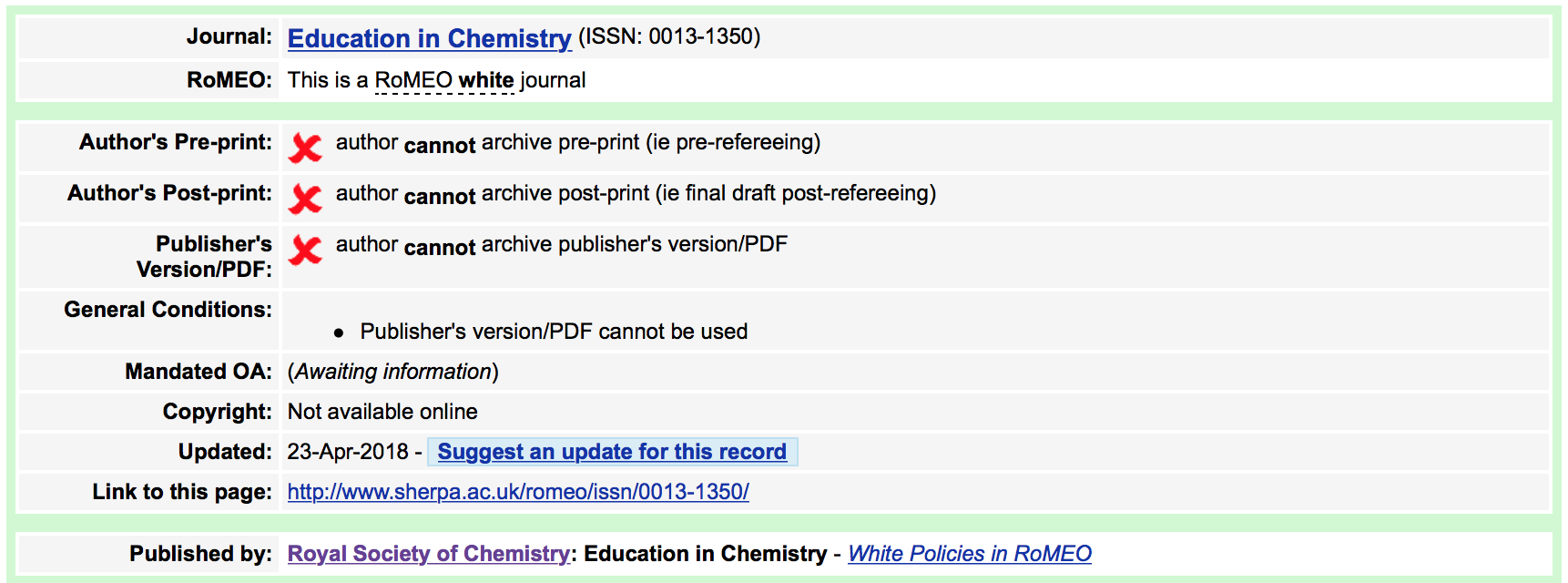In this detailed image caption, the information presented relates to a book and is enclosed within a rectangular frame, either white or green. At the top, the heading "Journal" is displayed in black text, followed by "Education and Chemistry" in blue text. Beneath this, "Romeo" is written in black text, indicating it is a Romeo white journal.

The first category, "Author's Preprint", features a red X on the right side with the message "Author Cannot Archive Preprint". The subsequent category, "Author's Postprint", also has a red X on the right with the statement "Author Cannot Archive Postprint". Moving on to "Publisher's Version/PDF", a similar red X indicates "Author Cannot Archive Publisher's Version/PDF". 

The section for "General Conditions" specifies that the "Publisher Version/PDF cannot be used". Under "Mandated OA", it states "Awaiting Information" in parentheses and notes that the "Copyright not available online". This was last updated on "23rd of April, 2018", with "Suggest an Update for this record" in blue text, underlined.

The final categories include a "Link to this page" with a provided URL address. Ultimately, the book is "Published by the Royal Society of Chemistry, Education and Chemistry" with "White Policies in Romeo" noted at the bottom.